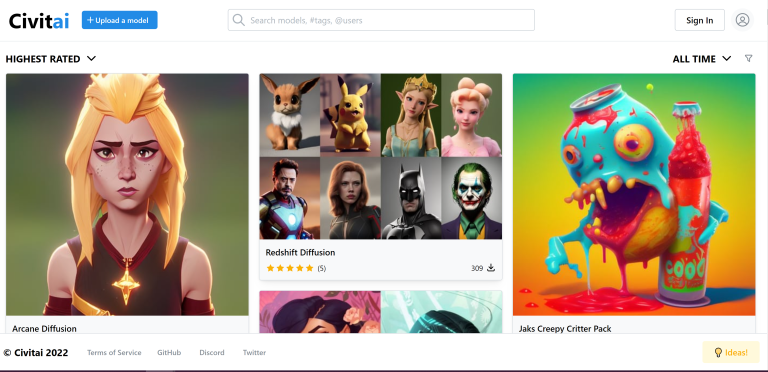Certainly! Below is the cleaned-up and detailed caption based on the provided description:

---

The image features a user interface with a white background. In the top left corner, there is the branding "CIVIT" in black and "AI" in blue. Below this, there is a prominent blue rectangular button labeled "Upload a Model". Adjacent to this button is a search box with the placeholder text "Search Models, Tags, and Users". To the right of the search box is a "Sign In" button and a default generic profile picture icon.

On the left side of the image, there is a section titled "Highest Rated," displaying a cartoon illustration of a person with long blonde hair, wearing a gold pendant shaped like a diamond at the end of a necklace. This illustration is labeled "Arcane Diffusion". To the right of this illustration, there is another section showcasing characters from various games, including Pokemon and Batman, under the label "Redshift Diffusion".

At the very bottom of the interface, there are links titled "Copyright Civitie 2022", "Terms of Service", "GitHub", "Discord", and "Twitter", indicating important legal and social media information about the platform.

---